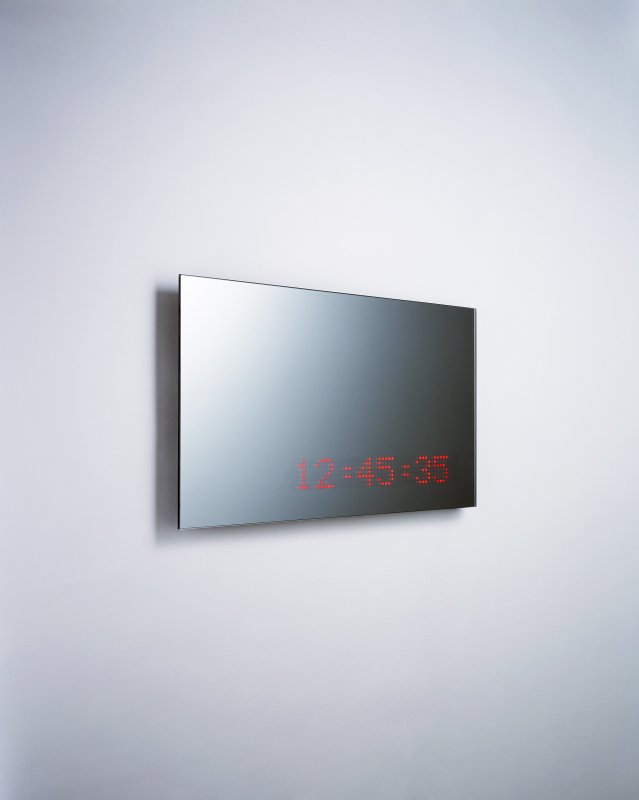The image depicts a minimalist setting with a primarily white wall featuring light gray gradients on the upper and lower sections. Centrally mounted on this wall is a rectangular screen, approximately five inches high and six inches wide. The screen exhibits a gradient from a bright upper left corner, reflecting a light source, to a darker bottom right corner, appearing almost black. The screen’s display is primarily gray, transitioning to black on the right side with a pronounced highlight in the upper left. Notably, the screen shows a sequence of red numbers—12:45:35—composed of small, red dots located in the lower right corner. The scene is simple, with no visible wires or surrounding electronics, emphasizing the screen as the focal point.